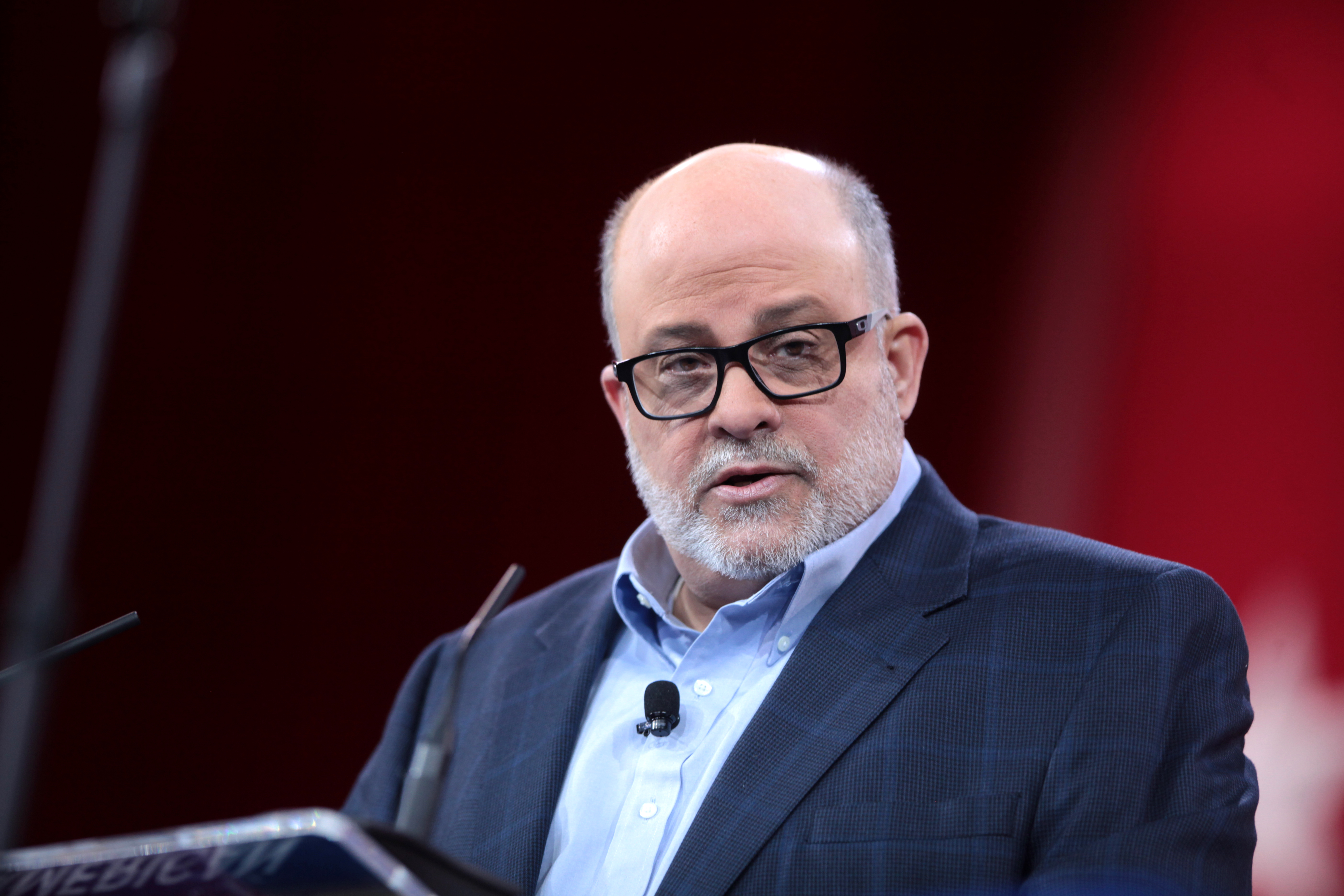This is a detailed photo of Mark Levin, the political commentator. He is standing near a podium adorned with a couple of thin black microphones. He also has a microphone pinned to his blue shirt, which is complemented by a blue suit, potentially checkered. Levin, an older white man, is identifiable by his thick black glasses and his facial hair: grayish-white, forming a mustache, goatee, and sideburns that skirt around his bald head. He is looking off to the center-right, although his body is slightly turned to the left. Behind him is a blurry red background, possibly a curtain, adding contrast to the image. The photograph is wider than it is tall.